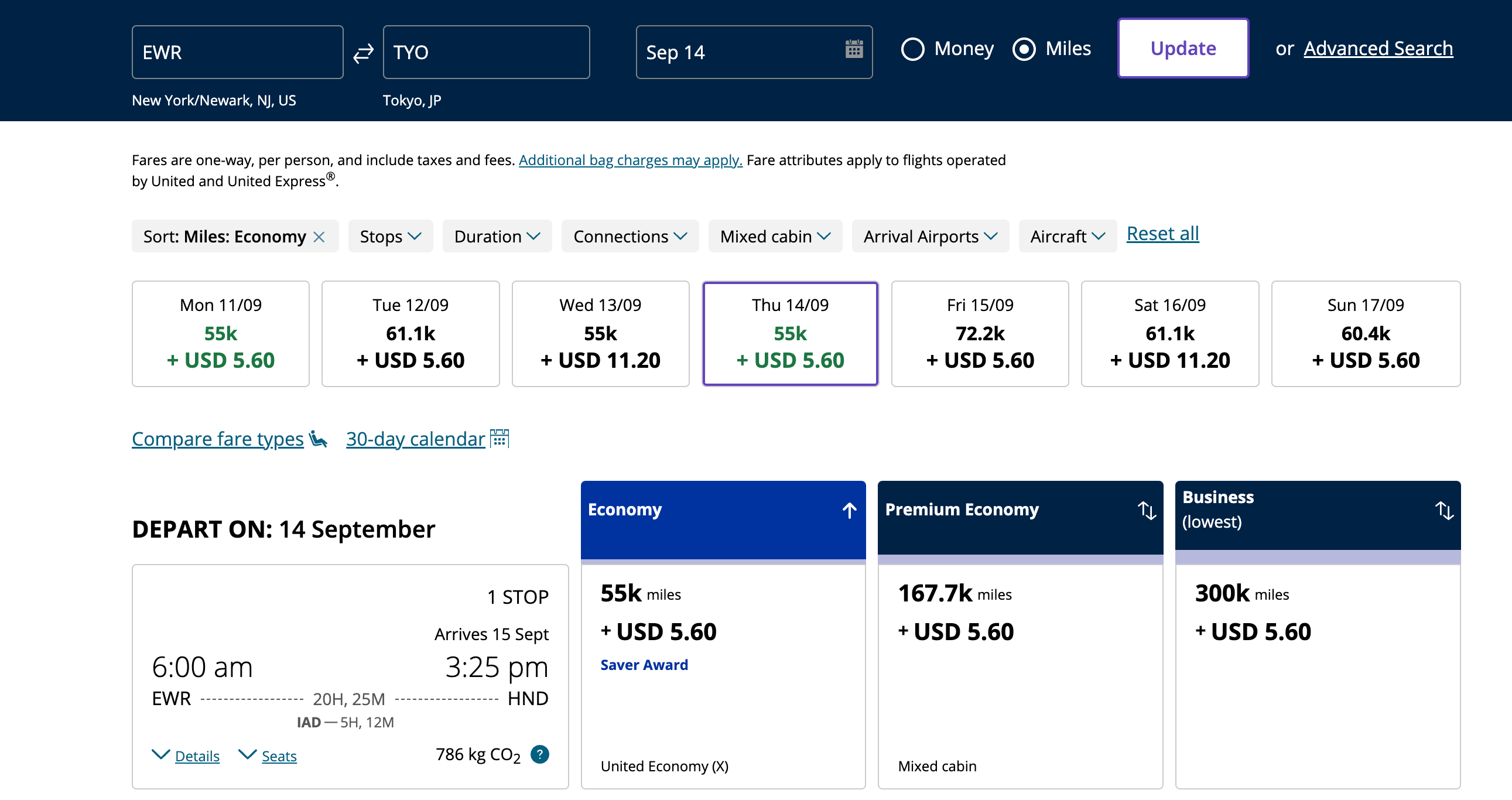At the top of the website, there is a navy blue header with white outlined text. This header section creates rectangular tabs with various travel details. The first tab reads "EWR," indicating Newark Liberty International Airport. Below, it specifies "New York/Newark, NJ, US." A bidirectional arrow suggests a round trip. The next tab shows "TKO," with "Tokyo, JP" written underneath, representing Tokyo, Japan.

The following section displays "SEP - September 14th" and includes financial and mileage details. A rectangle with a white background and a purple border contains the options "Update" in purple and "Advanced Search" in white, underlined.

Below this are additional details written on a white background. It mentions that fares listed are one-way per person, inclusive of taxes and fees, with a note in blue stating "Additional bag charges may apply." Another line in black reads, "Fare attributes apply to flights operated by United and United Express," followed by various filter options like miles, economy, stops, duration, connection, mixed cabin, arrival at airports, and aircraft. A blue text option "Reset all" is available for clearing selections.

The flight date options start with "Monday 11/09," marked at "55K in green plus USD 560." The subsequent days list similar details: Tuesday shows "61.1K plus USD 5.60," followed by identical pricing for the night. Thursday lists "55K," Friday "72.2K," Saturday "61.1K," and Sunday "60.4K."